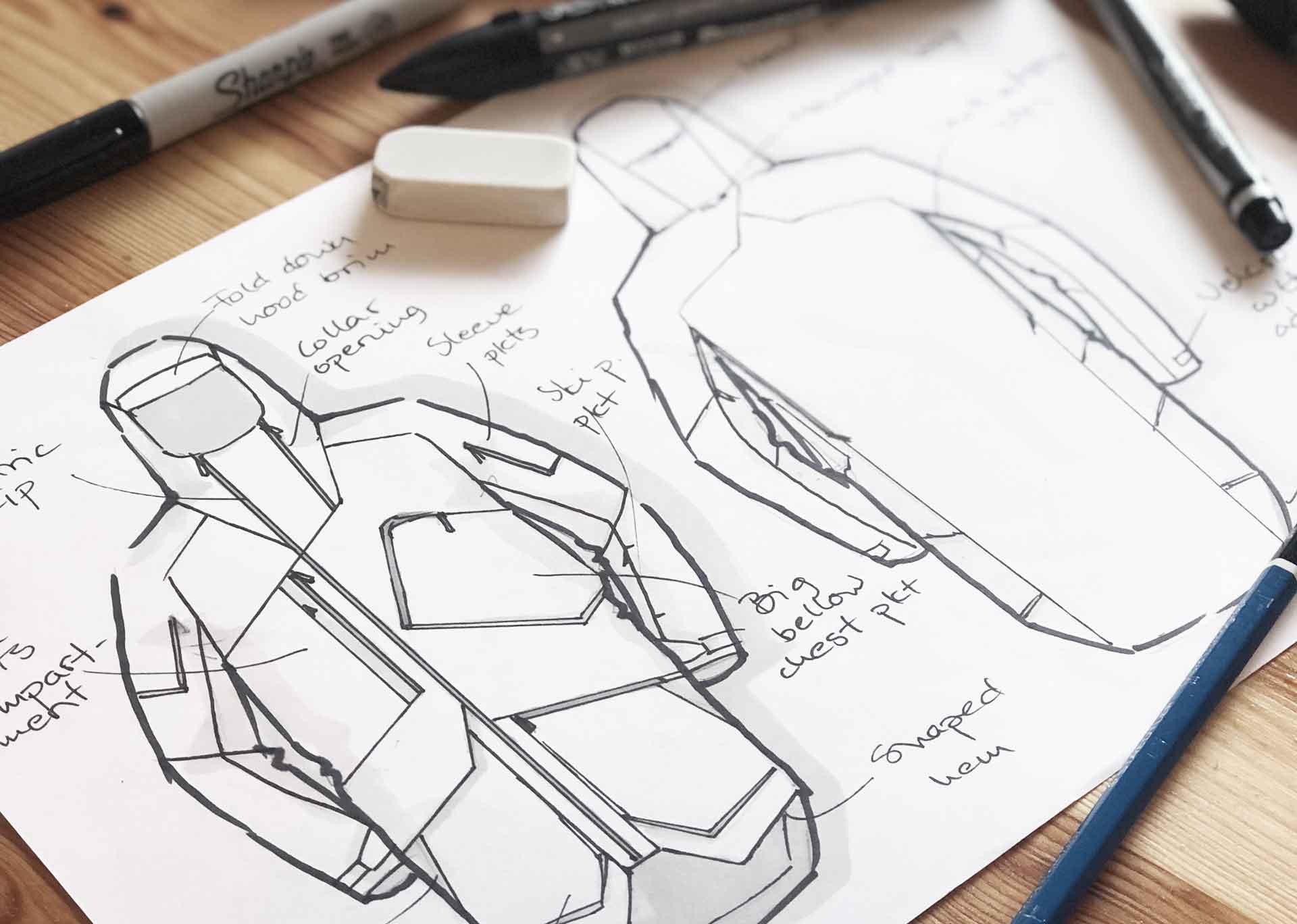This color photograph captures a detailed sketch of a raincoat laid out on a brown wooden table, viewed from above. The sketch, executed in black ink on a large white sheet of paper, presents both the front and back views of the coat. Surrounding the paper are various drawing tools—a black Sharpie in the upper left corner, a blue pencil, a black pen, and a white eraser—scattered across the desk surface, whose wood grain is just visible. The raincoat design features intricate labeling, with lines pointing to various parts of the garment. Among the readable handwritten notes are descriptors like "fold-down wood brim," "collar opening," "sleeve pockets," "big bellow chest pocket," and "shaped hem," indicative of a functional, long-sleeved jacket with large pockets and a hood. The meticulous annotations suggest a detailed design process, possibly for a sturdy outdoor garment.